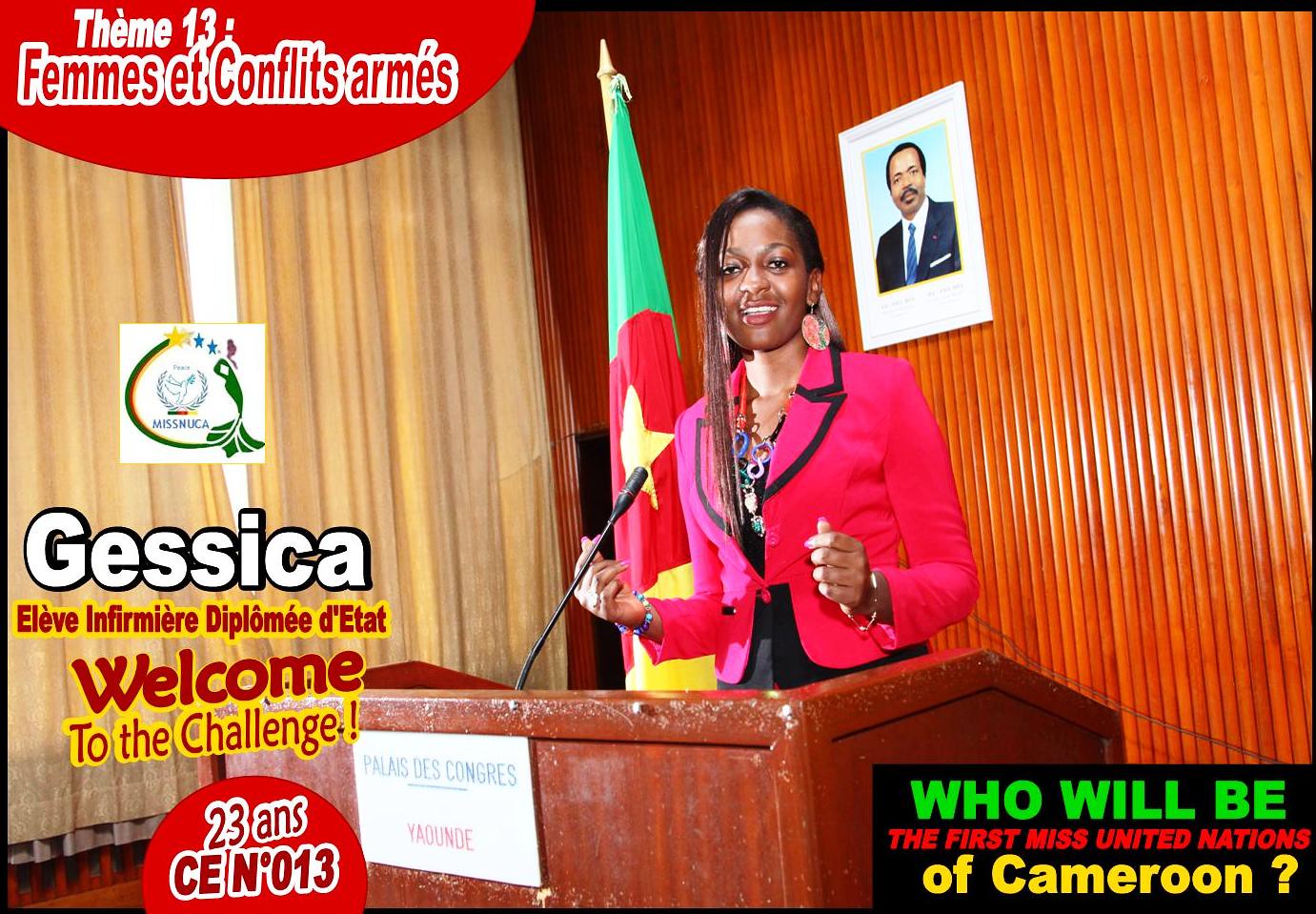The image depicts a young woman from Cameroon standing at a podium adorned with a black microphone. She is wearing a striking pink suit with black trim on the collar, and a dark dress underneath. Her long black hair is intricately braided, and she accessorizes with earrings, necklaces, and bracelets. Her poised stance is set against a wooden backdrop featuring a portrait of a man in a suit and blue tie. To her right is the flag of Cameroon.

Prominently, the upper left corner of the image bears the inscription "Team 13 Femmes et Conflicts Arms," followed by the name "Gessica," along with the titles "Élève Infirmier Diplôme de l'État," and "23 ans," indicating she is 23 years old. Additionally, a bright banner reads, "Welcome to the challenge."

The lower right corner of the image poses an intriguing question, "Who will be the first Miss United Nations of Cameroon?" In the lower left, further text includes the phrase "Palais des Congrès Yaoundé," distinguishing the location, with "Palais des Congrès" in blue and "Yaoundé" in red. Overall, the scene appears to be an advertisement or campaign photo, emphasizing Gessica's candidacy amidst a formal and supportive setting.